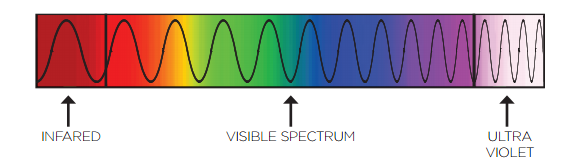The image is a detailed light spectrum diagram presented as a thin, rectangular bar that transitions smoothly from red on the left to white on the right through the colors of the rainbow—red, orange, yellow, green, blue, and purple. A black, wavy line runs across the length of the bar, starting with wide, spaced-out waves on the left and becoming increasingly closer and tighter towards the right. At the red section on the far left, an upward-pointing arrow labeled "infrared" is present. In the central part of the diagram, between the green and blue sections, there is another upward-pointing arrow labeled "visible spectrum," corresponding to the vibrant rainbow colors. Finally, at the far right end where purple transitions to white, an arrow labeled "ultraviolet" is positioned. The descriptive elements capture the entire range of the color spectrum and delineate the infrared and ultraviolet regions beyond human visual perception.